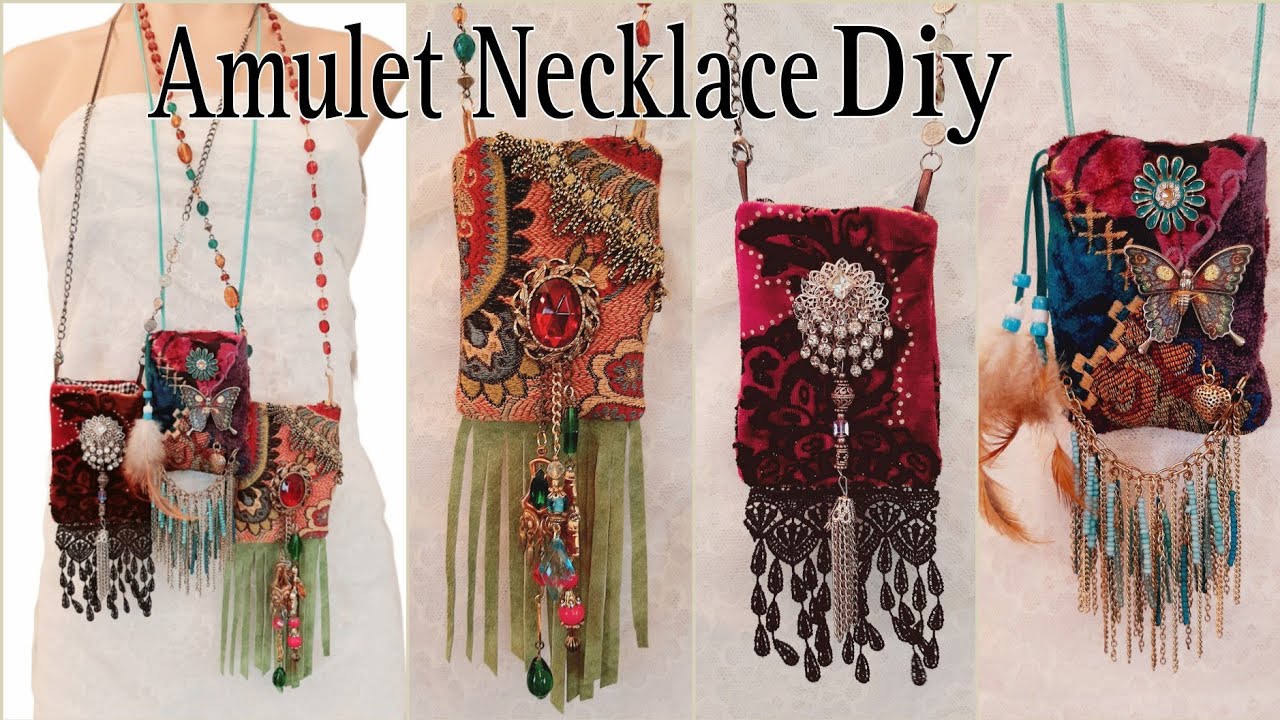This detailed image caption captures the repeated and shared elements from each description:

The image features a horizontal advertisement titled "Amulet Necklace DIY" with a central bold text. It is divided into four sections: the first frame shows an armless mannequin dressed in a white outfit, adorned with three large amulet necklaces that resemble small pouch-like purses. Each amulet hangs from the neck and is embellished with beads, tassels, and trimmings. The first amulet features silver-like and beaded trimmings, the second includes green beads, and the third incorporates fabric elements in its design. The other three sections provide close-up views of each individual amulet, highlighting their intricate details and vibrant colors which include reds, oranges, deep olive green, black, brown, and some blue. The amulets are designed with various jewels, feathers, and long hanging tassels, emphasizing their elaborate craftsmanship and decorative nature.